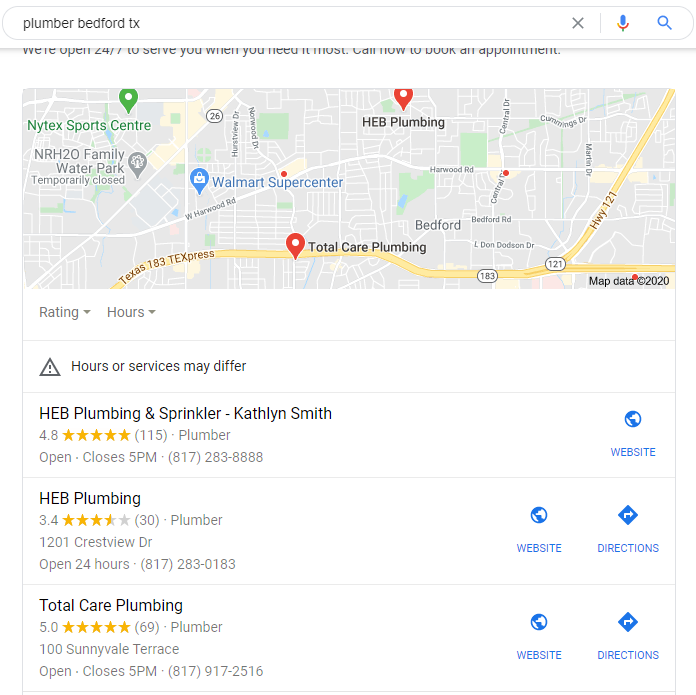The image displays a search bar with the query "Plumber, Bedford, Texas" entered. An 'X' icon is present to the right, allowing the user to clear the search bar. A microphone icon is integrated within the magnifying glass symbol, indicating voice search capability. Below the search bar, a map features several pinpoint markers denoting the locations of various plumbers. A warning icon, a triangle with an exclamation point, is present with a message stating "Hours or services may differ."

Below the map, the search results begin with:

1. **H.E.B. Plumbing and Sprinkler - Kathleen Smith**
   - Rating: 4.8 stars from 115 reviews
   - Status: Open now, closes at 5 PM
   - Links: Website and phone number available

2. **H.E.B. Plumbing**
   - Rating: 3.4 stars from 30 reviews
   - Address: 1201 Crestview Drive
   - Links: Website and directions available

3. **Total Care Plumbing**
   - Rating: 5 stars from 69 reviews
   - Status: Closes at 5 PM